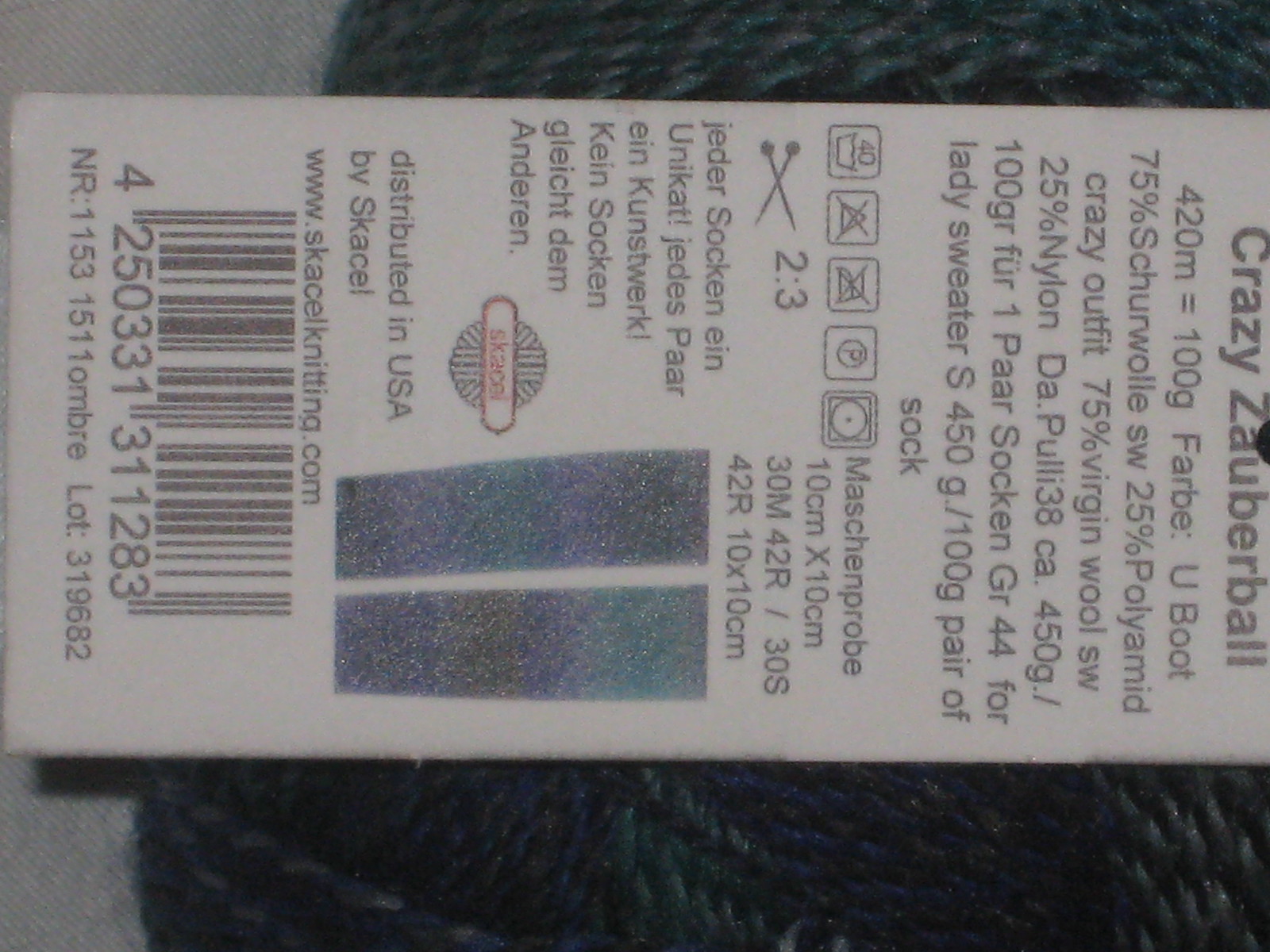This image features a sideways photograph of a product tag resting on a background of dark blue, turquoise, and grey yarn. The tag, made of cardboard, occupies the majority of the image with its top located to the right side due to its 90-degree rotation. Prominently written at the top of the tag is "Crazy Zauberball." Below this, detailed product information includes “420m equals 100g” and fiber content such as “75% Virgin Wool SW, 25% Nylon.” Additional text is primarily in German, alongside care instructions indicated by laundry symbols. At the bottom of the tag, it states "Distributed in the USA by SkateSkill" and features a large barcode with a serial number. The surrounding yarn, with its dark blue and turquoise hues, is partially visible behind the tag, enhancing the visual context of the product.